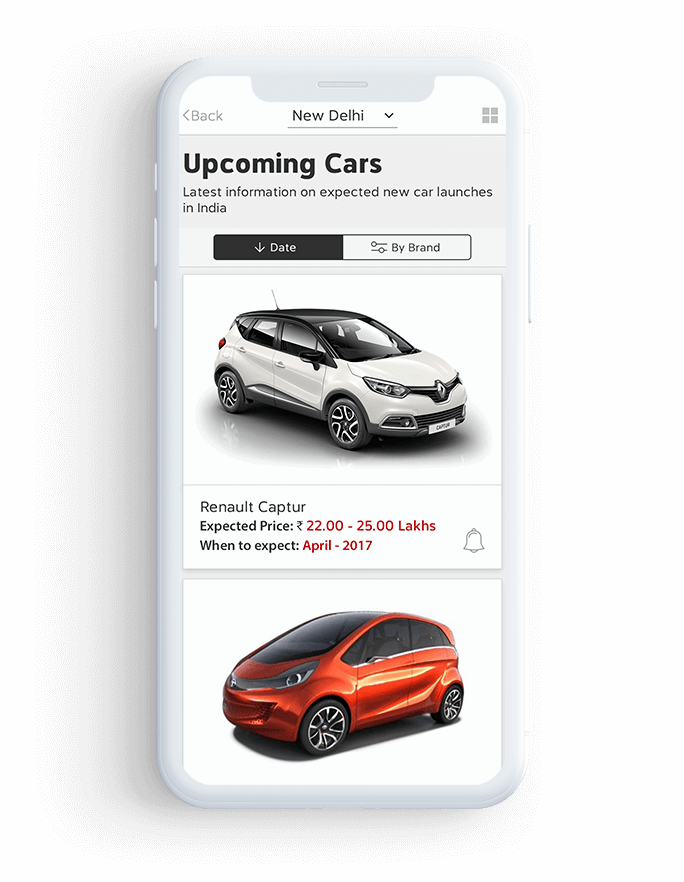The image appears to be a screenshot from a mobile device, specifically showcasing an interface reminiscent of the Carvana app or website. The majority of the background is white, providing a clean and minimalist look.

At the top of the image, there is a white navigation bar. On the left side of this bar, there is a gray back button with an arrow pointing to the left. On the right side, there are four gray squares arranged in the shape of a larger square, presumably functioning as a toggle button to switch between grid and list views of the inventory.

In the center of the top bar, "New Delhi" is displayed in black font alongside a drop-down menu, indicating that users can change their search location.

Directly below the navigation bar is a section with a light gray background and bold, capitalized text that reads "Upcoming Cars." Underneath this title, there is a subheading stating "Latest Information on Expected New Car Launches in India."

Beneath the gray section, there is a black button with white text that reads "Date" with a downward arrow, signifying that the cars are sorted in ascending order by date. Adjacent to this date-sort button, there is a filter button that allows users to filter the results by brand.

The main content below these controls features images of cars. The first visible car is white, while the second one is orange, each presumably representing upcoming car models available for view.